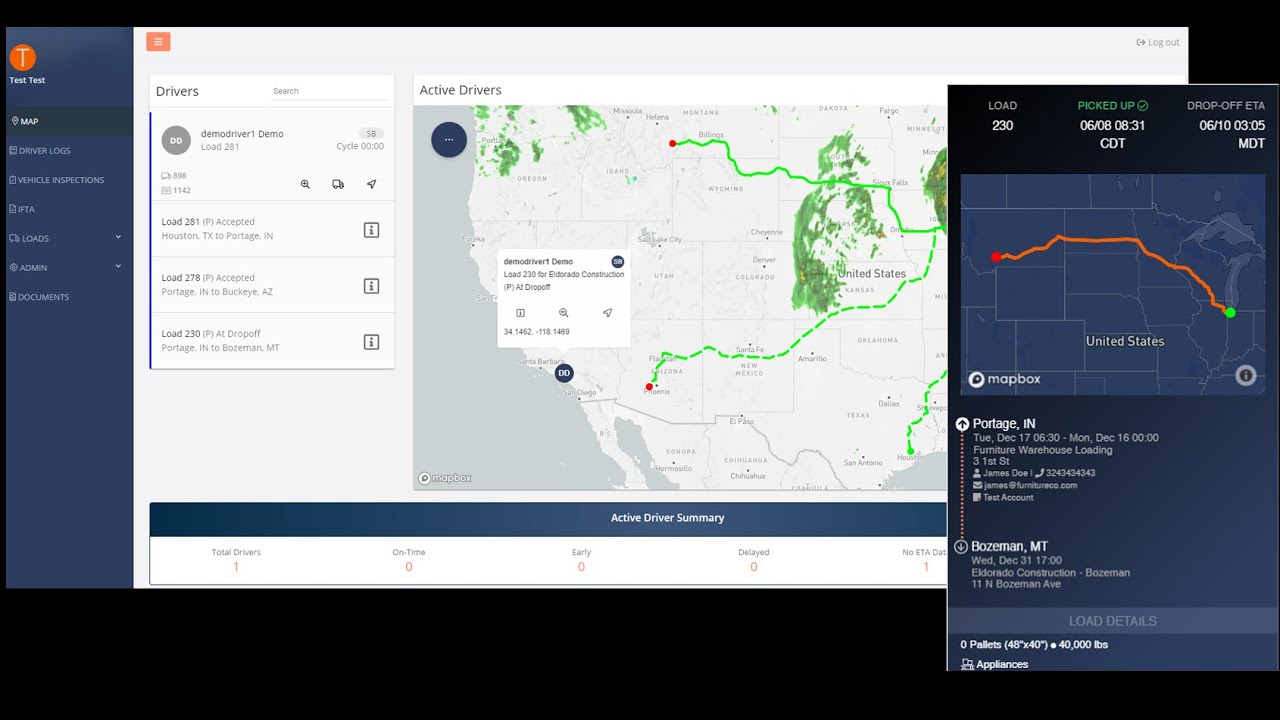The image depicts a website dedicated to drivers, possibly truck drivers, showcasing a map of the western United States adorned with green lines that likely represent roads. To the left of this map, a prominent white square labeled "Drivers" occupies the top left corner. Beneath this label, the word "Load" appears three times, each instance accompanied by numerical figures, which probably denote the loads that truck drivers are transporting along this route. In the bottom left corner of the map, the phrase "Active Drivers" is displayed, accompanied by a smaller square providing details about a specific active driver. Additionally, a portion of the Midwest is visible to the right of the main map, highlighting two key locations: Portage, Indiana, and Bozeman, Montana. An orange line connects these two cities, both of which are distinguished by white lettering.